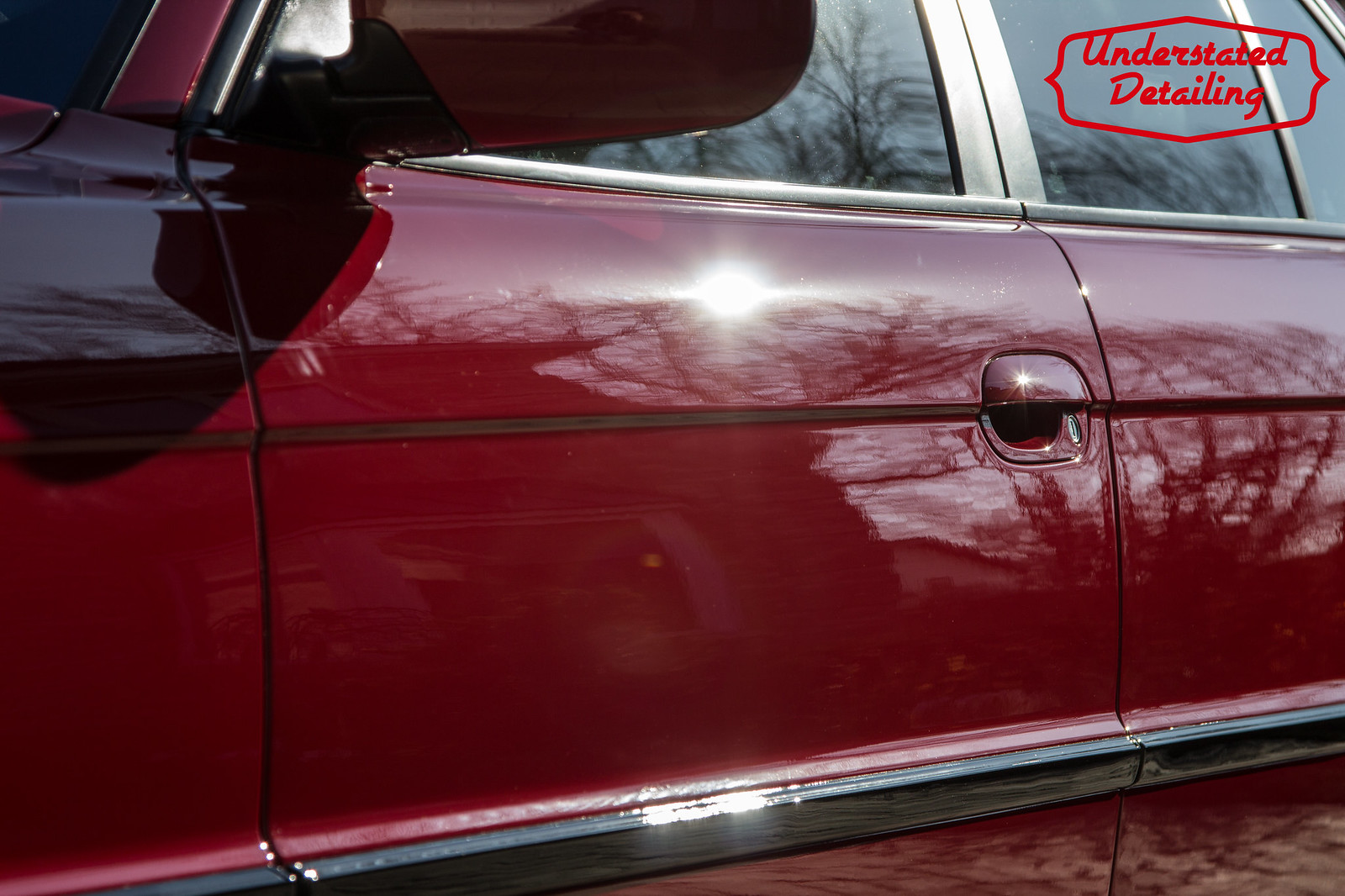This photograph, taken in landscape orientation, features a close-up view of a substantial, four-door burgundy car with a shiny, dark blood red finish. The focus is on the driver's side door and mirror, highlighting the recessed door handles that match the burgundy body panels. A silver, horizontal chrome stripe runs the length of the lower portion of the doors, complemented by chrome trim around the windows. The image, captured outdoors during daylight hours, reveals reflections of bare trees on the car's sleek surface and shimmering windows, suggesting it might be winter. In the upper right corner, the logo "Understated Detailing" is prominently displayed inside a red, fancy box or bubble design, indicating this car has been meticulously cleaned and is being showcased by a detailing company.